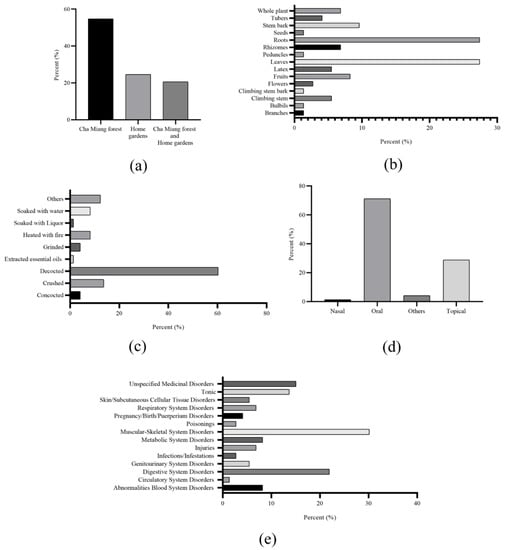The image displays a series of detailed bar charts labeled A through E, set against a white background. Each chart consists of dark black and gray bars, and they all feature both an X and Y axis. There are five charts in total, arranged with two on the top row, two in the middle, and one at the bottom. Although the text is quite blurry and difficult to read, some labels such as "whole plants," "leaves," "flowers," "bark," and possibly "bleachers" or "beaches" can be discerned on the charts. Chart A presents a prominent large black bar alongside two smaller gray bars. Chart B seems to have multiple bars, with two large ones standing out. Chart C also features several bars with one particularly long one. Chart D is distinguished by one large gray bar among smaller ones. Chart E contains multiple labeled items on the left with corresponding bars extending to the right. Despite the difficulty in reading the exact text, the visual arrangement and color coding of the bars are clear.